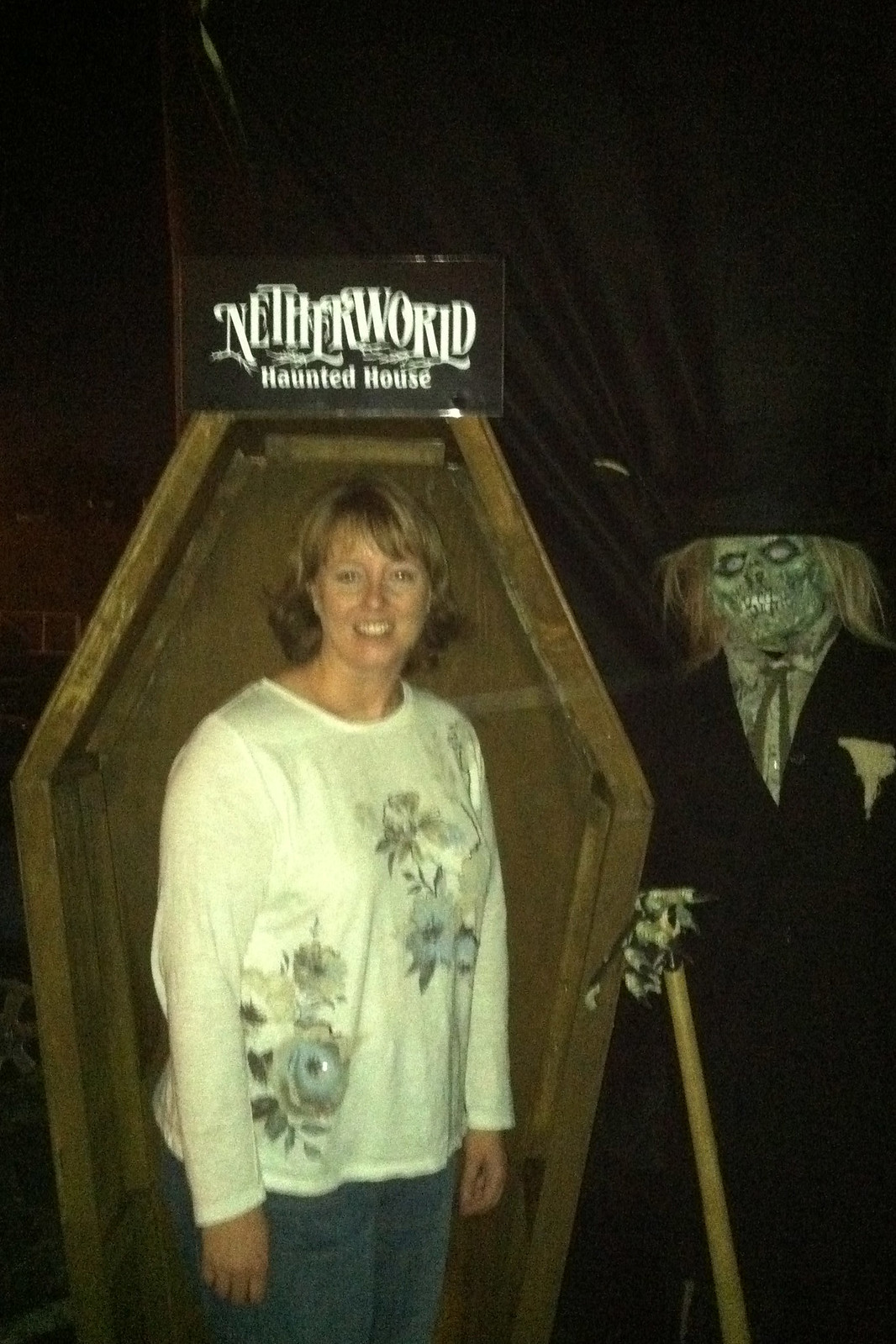The photograph captures a middle-aged white woman, likely in her 30s or 40s, standing in front of an open wooden coffin with a black sign on top that reads "Netherworld Haunted House" in white letters. She has short blonde hair that doesn't reach her shoulders and is dressed in a white long-sleeve shirt adorned with flowers paired with blue jeans. The woman is smiling and looking directly at the camera. Positioned to her right is a creepy, Crypt Keeper-like Halloween prop dressed in a black suit, tie, and hat, holding a cane, and grinning with sharp teeth. The entire scene is set against a backdrop of a black curtain, suggesting a haunted house setting. The colors in the image predominantly include various shades of green, black, white, blue, and brown.